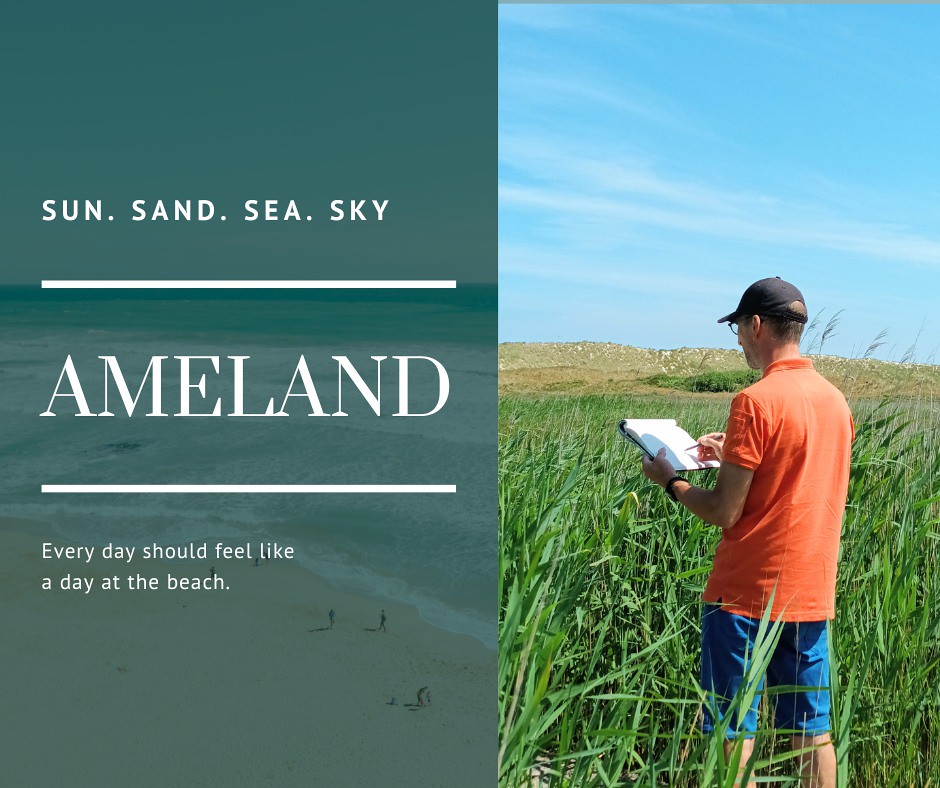The image is divided into two panels. On the right side, a man is standing in a field with tall green grass, featuring a high beach dune in the background against a clear blue sky with wispy clouds. He is dressed in an orange polo, a black baseball cap, and knee-length blue shorts. He holds a white notepad in his left hand and writes with a pencil in his right hand, his left wrist adorned with a black watch. Meanwhile, on the left side, a translucent teal rectangle overlays a photo of a sandy beach with five people and the ocean in view. The text in white letters reads, "Sun, Sand, Sea, Sky, Ameland." Below a separating line, it continues, "Every day should feel like a day at the beach."